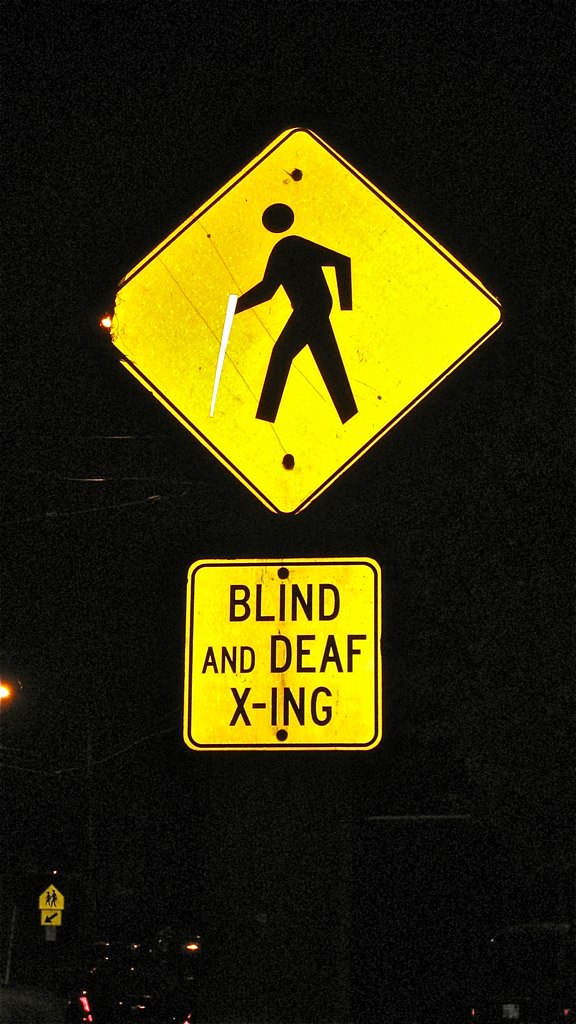This photograph, taken at night with a very dark background, captures a highly reflective yellow road sign, prominently featuring a black icon of a person walking with a white cane, indicating it's a blind and deaf crossing. The sign's main part is a large diamond shape with a black border. Beneath it, there's a smaller yellow square sign also with a black border, bearing the text "BLIND AND DEAF X-ING" in black. In the background, faint car lights and another road sign are visible. This distant sign appears to depict a parent and child, with an arrow pointing to the lower left beneath it, suggesting a school crossing area. The presence of this specialized signage indicates a heightened safety measure, possibly near a school for the blind or a relevant governmental building.